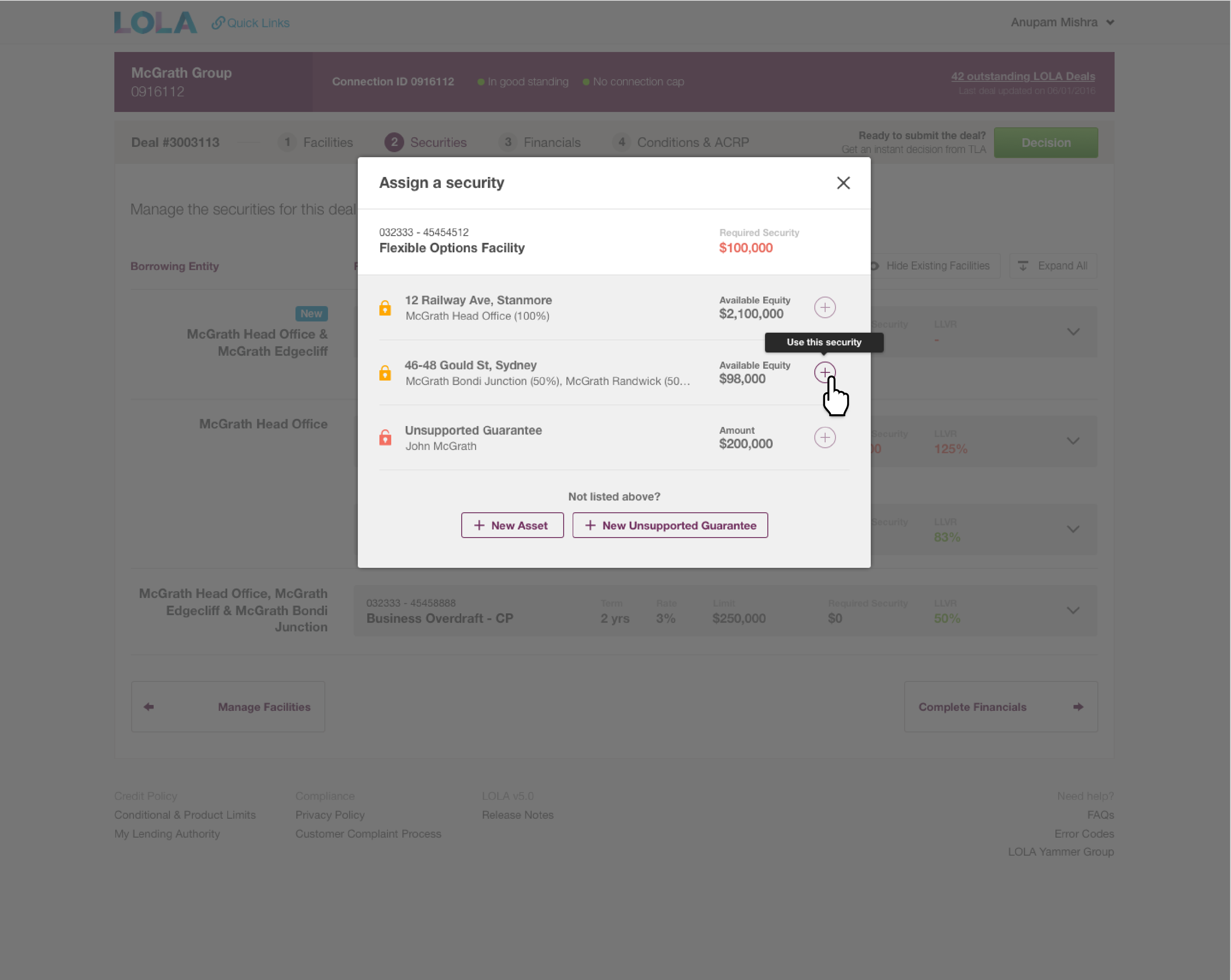Here is a detailed and cleaned-up caption for the image:

---

The screenshot displays a website page overlaid by a central pop-up window for assigning a security, which is slightly elevated in the frame. The pop-up has a white background at the top, featuring a dark gray heading that reads "Assign a Security," accompanied by a gray 'X' icon on the far right for closing the window.

A thin gray line separates this header from the subsequent section, which is also set against a white background. On the left, there are two lines of text. The first line, in medium gray, displays "032333-45454512," and directly below it, in bold text, is "Flexible Options Facility." To the right of this, light gray text indicates "Required Security," with an adjacent red text stating "$100,000."

The rest of the pop-up has a gray background. The first row features an orange lock icon, followed by bold text stating "12 Railway Ave, Stanmore." Beneath this is light gray text reading "McGrath Head Office (100%)." To the right, it notes "Available Equity, $2,100,000." Further right, we see a faded purple circle containing a plus sign.

The second row follows a similar format, showcasing a lock icon and featuring "46-48 Gold Street, Sydney" in bold. Beneath it, in parentheses, are "McGrath Bondi Junction (50%)" and "McGrath Randwick (50%)." The available equity here is $98,000, and to the right is a darker purple circle with a plus sign, accompanied by a black speech bubble with white text that says "Use This Security." A white hand-shaped cursor with a black outline hovers over this button.

The final row includes a red lock icon and the text "Unsupported Guarantee." To its right, the text reads "John McGrath," with an amount listed as "$200,000." Another faded purple symbol sits to the far right.

The webpage behind the pop-up is partially visible but dimmed to emphasize the pop-up window.